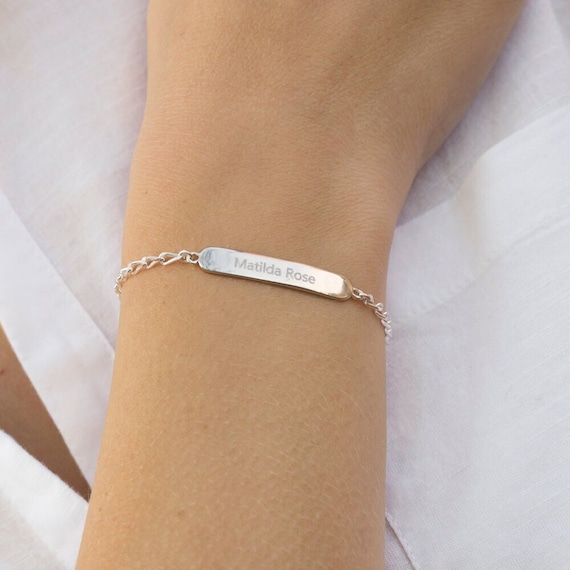The photograph showcases the right hand of a white person wearing a silver chain bracelet. The bracelet features a rectangular-shaped silver pendant with the inscription "Matilda Rose." The hand is positioned across the person's left chest, against a white, thin, and slightly open pocket button-down dress shirt. The fingers are not visible, extending out of the top of the image, while the wrist remains the central focus. The background consists solely of the white shirt, highlighting the simplicity and elegance of the scene.